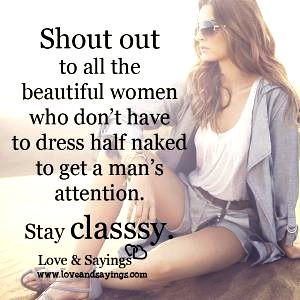In the image, a young woman with long, flowing dark hair and sunglasses sits casually on the sand, basking in the sunlight. She sports a white tank top underneath a loose-fitting blue-grey button-down shirt and short shorts. The photograph exudes an effortless, laid-back vibe. Overlayed on the left side of the image is a bold message: "Shout out to all the beautiful women who don't have to dress half-naked to get a man's attention. Stay classy." The word "classy" is highlighted in bold black text, reinforcing the sentiment. At the bottom of the graphic, the source is credited as "Love and Sayings" with their logo featuring two interlocking hearts and the URL "www.loveandsayings.com," suggesting it's an advertisement for the website where personal sayings can be created and shared.